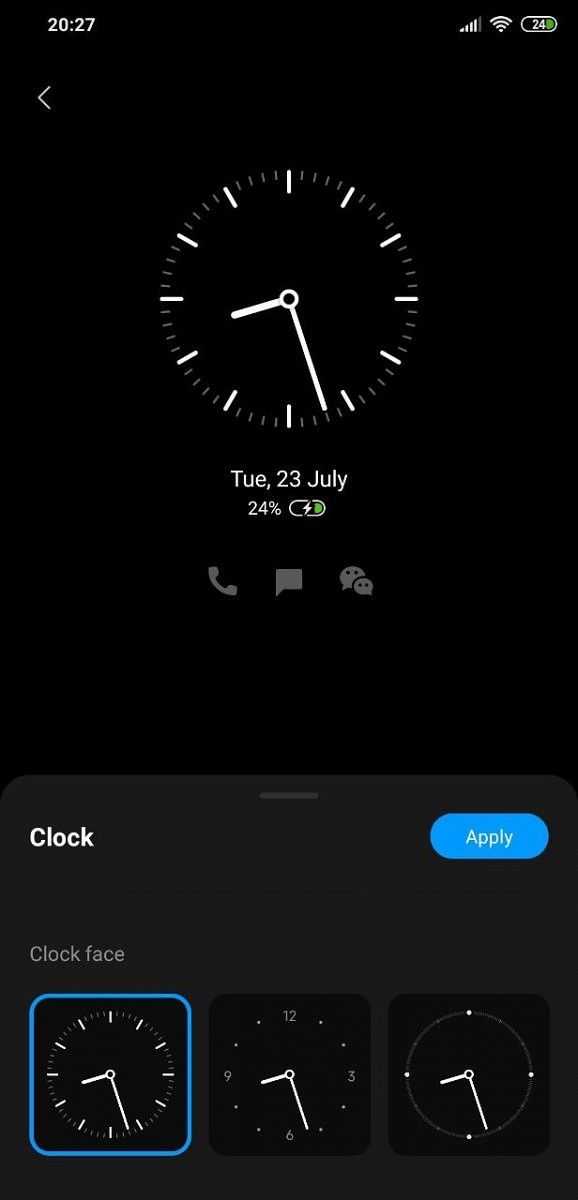In the image, the top section indicates a nearly full battery, specifically at 24%, with a timestamp suggesting the status as of Tuesday, July 23rd, 2027. The background features an oval-shaped clock with a blue face, marking the hours of 12, 3, 6, and 9. A gray clock overlay highlights the same hours with prominent shorthand and big hand indicators. The interface includes options to like and comment, as well as a visible comment section at the bottom. The word "apply" is also present, suggesting an actionable prompt within the image context.